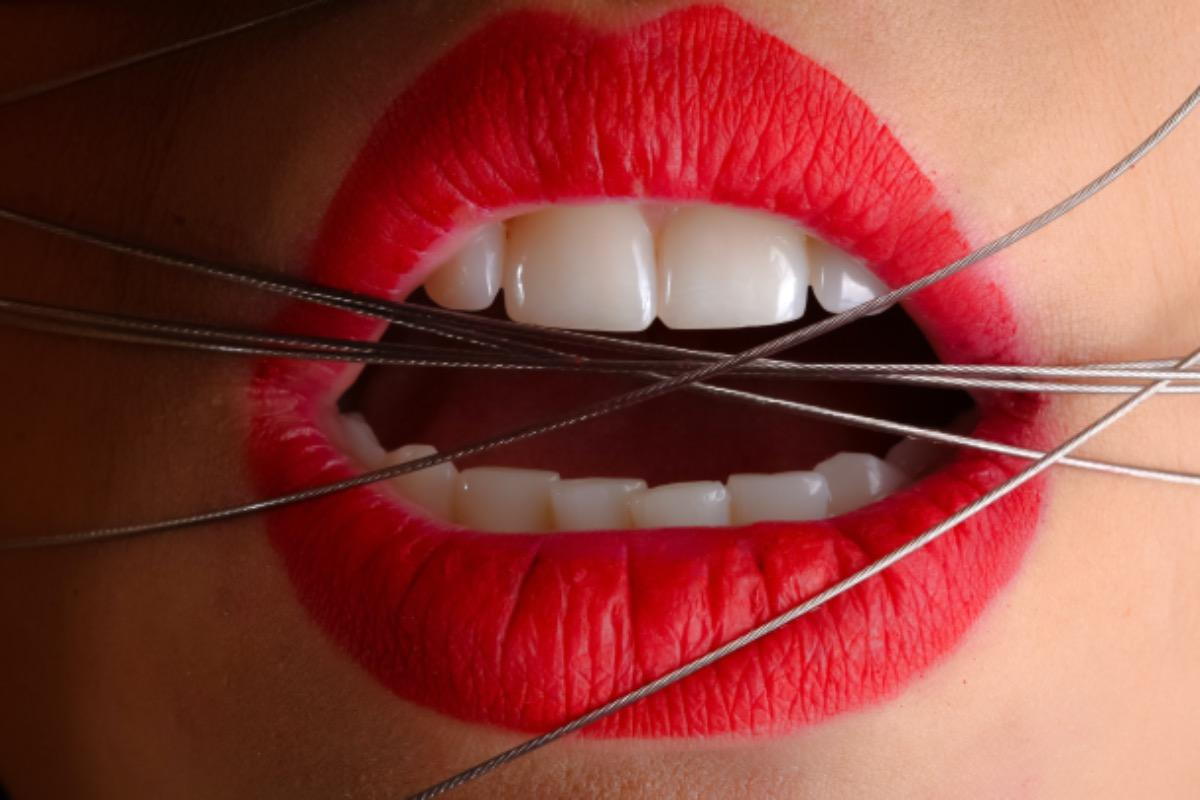A close-up of a woman's mouth showcases her striking bright red lipstick, accentuating her slightly parted lips. Her impeccably white teeth are visible, with both her upper and lower front teeth prominent. Intricately crisscrossing across her lips and face are several thin, silver-colored wires. Two wires, starting from the lower left side, stretch upward to the right side of her mouth, while four more wires, bundled closer together, traverse from the right side to the left, arching over her lips. Her partially visible tongue and the tension of the wires highlight the focus on her vividly red lips and the intricate interplay of the metallic threads.